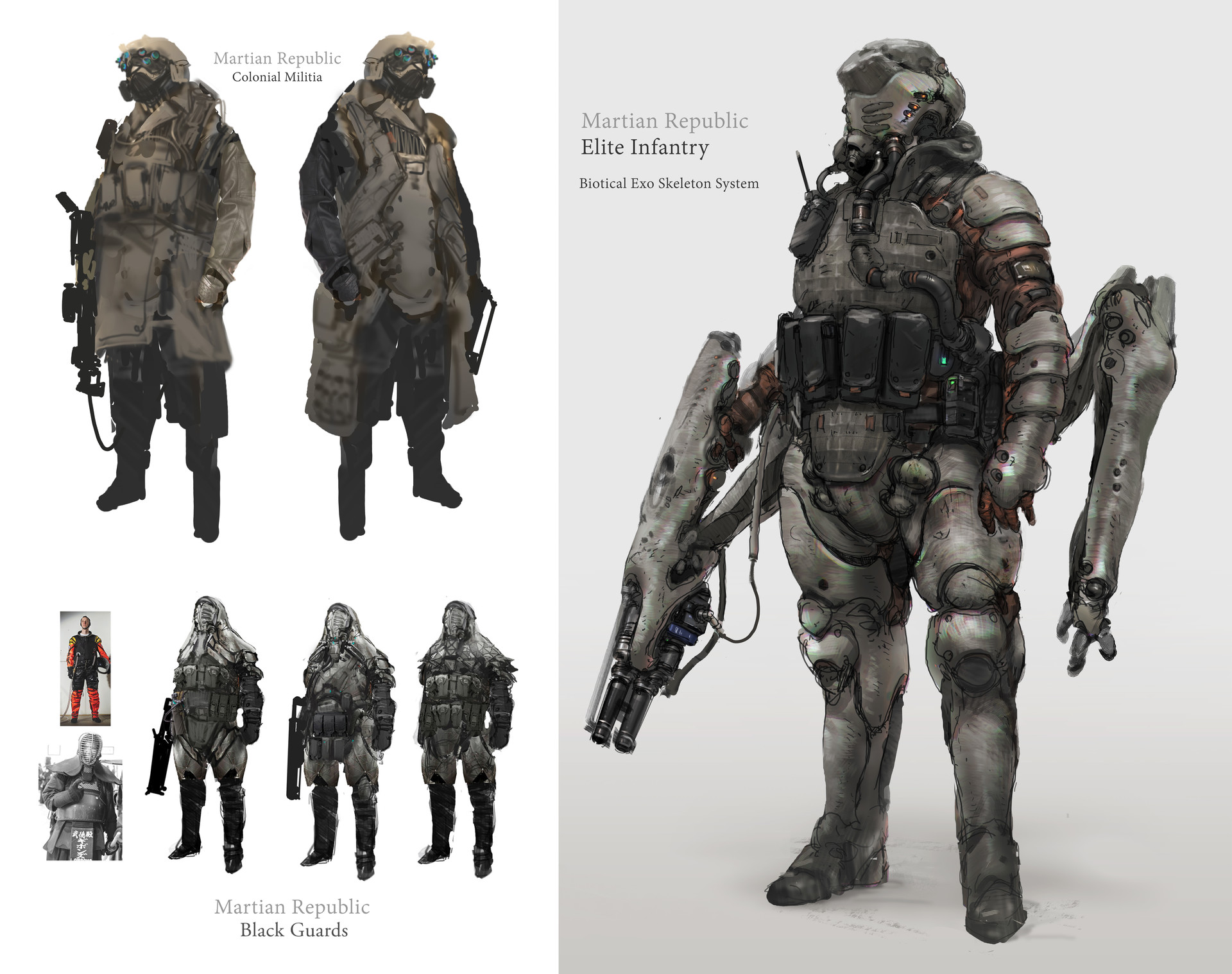The image depicts a detailed rendering of futuristic soldiers labeled as part of the "Martian Republic." Dominating the right side is a larger figure identified as the "Martian Republic Elite Infantry," clad in heavy armor with a helmet and mask, and is equipped with a massive gun. This character features a Bio-Attical Exoskeleton System with additional mechanical arms extending from its back. The background is gray, highlighting the robust and imposing nature of the figure. On the left, there are several smaller views of similarly armored characters, categorized as "Martian Republic Colonial Militia" at the top and "Martian Republic Black Guards" at the bottom. These figures, although a bit smaller, share the same militaristic and heavily-armored appearance, dressed in black and gray suits, and are equipped with various weapons, indicating their readiness for battle. The scene portrays a formidable and well-equipped futuristic military force designed for combat efficiency.